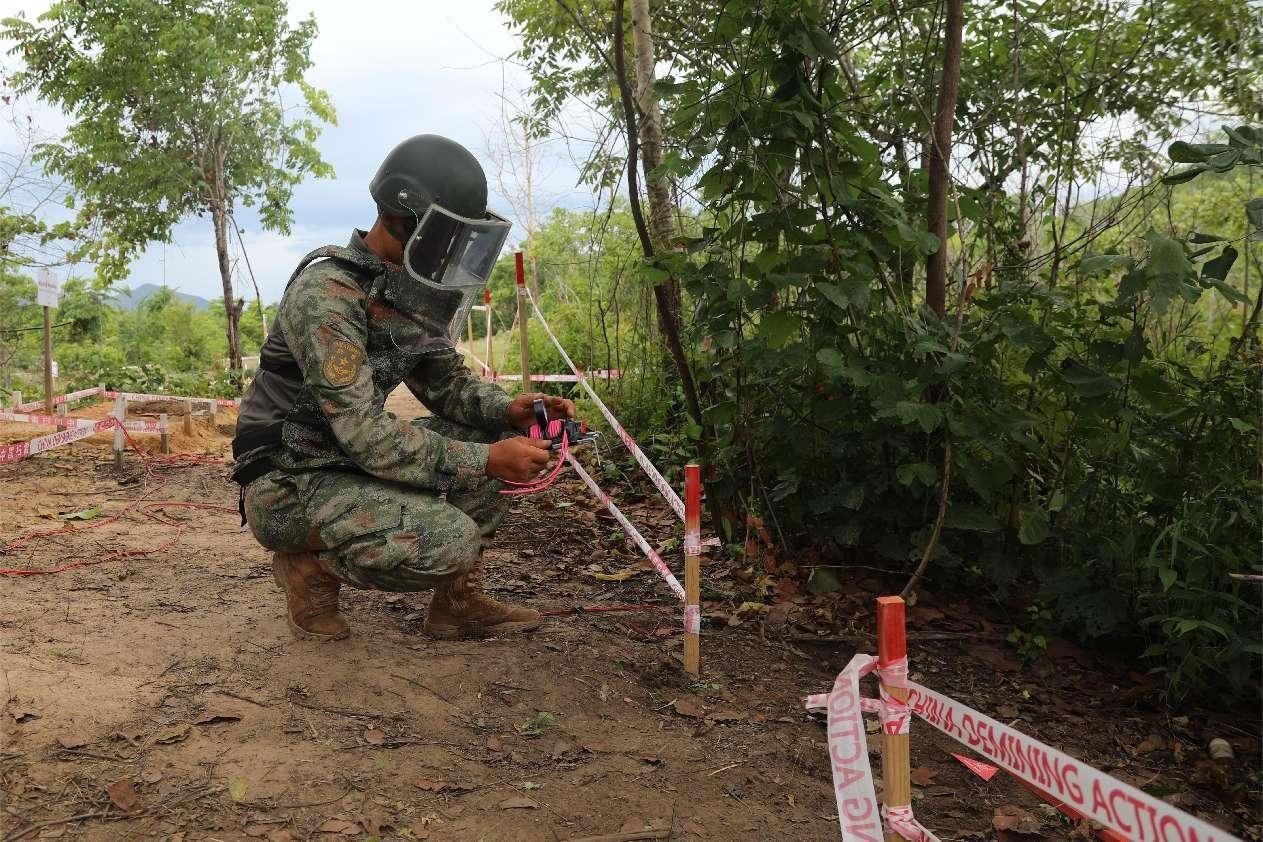In this high-quality, daytime photograph, we see a young person wearing military fatigues, brown boots, a helmet, and a thick glass face shield, crouched down on a dirt path in a wooded area. Surrounded by foliage, the individual, who appears to be dark-skinned, is intently examining an object in their hands that resembles a spool with pink ropes. The area is cordoned off with banners wrapped around wooden poles, displaying text that reads "Demining Action." The scene suggests that the person is engaged in a demining operation, likely scanning for landmines. In the background, a grassy expanse with trees and bushes extends towards a distant mountain under a partly cloudy, blue sky.